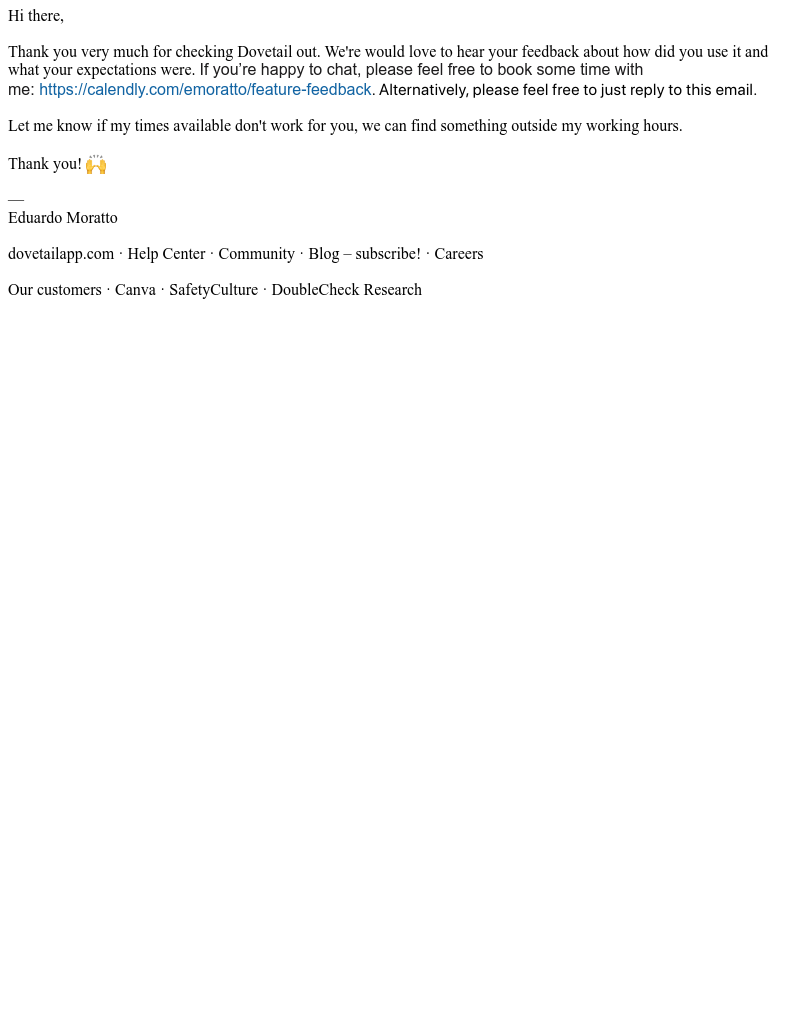This image depicts a digital message formatted as an email. At the very top, in black print, it begins with the greeting "Hi there," followed by a space. Aligned to the left, the message continues with, "Thank you very much for checking Dovetail out." 

The email then proceeds to express an interest in receiving feedback, stating, "We would love to hear from you and your feedback about how you used it and what your expectations were." It invites recipients to schedule a conversation, saying, "If you're happy to chat, please feel free to book some time with me," and includes a clickable HTTPS link for scheduling.

Alternatively, the message suggests, "...please feel free to just reply to this email." In a subsequent paragraph, the sender offers flexibility in scheduling, stating, "Let me know if my available times don't work for you, we can find something outside my working hours."

The email closes with a heartfelt "Thank you!" followed by a clapping hands emoji. Beneath this closing, the sender's name, Eduardo Moranto, is presented, accompanied by additional websites and contact information.